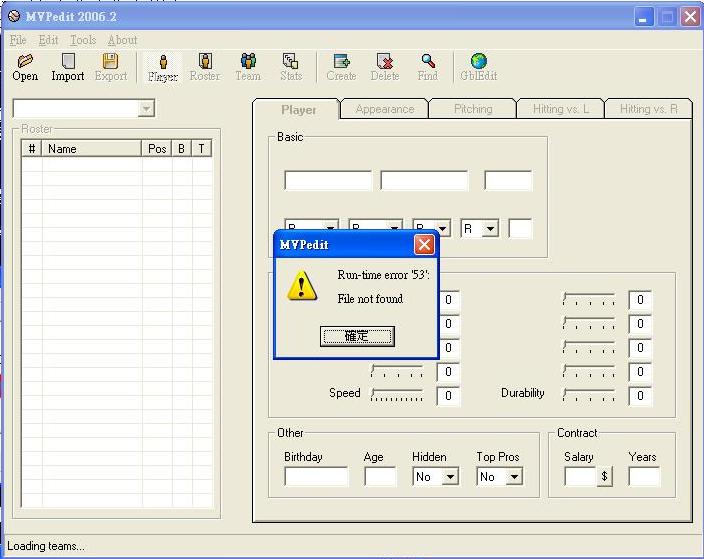The image is a detailed screenshot of an older computer application named MVPedit 2006.2, displayed within a light blue-bordered window. The interface itself is light gray, featuring multiple sections and icons typical of a Windows operating system. At the very top, the application name is highlighted with a blue background, and the standard Minimize, Maximize, and Close (X) buttons are located in the upper right corner.

Beneath the title bar, the menu includes options like File, Edit, Tools, and About, followed by icons for actions such as Open, Import, Export, and several others, including Flyer, Roster, Team, Stats, Create, Delete, Find, and GBL Edit. Below these icons, the interface contains menu items and grids designed for data entry, though the fields are currently empty.

Centered on the screen, an error message box stands out with a blue outline and a blue bar at the top, containing a red X in the upper right corner and a yellow warning triangle with an exclamation mark. The title of this pop-up reads "MVPedit Runtime Error 53: File Not Found." Below this message is a button labeled in Asian characters. Partially obscured by the pop-up are sections focused on defining player attributes like Player Appearance, Pitching, Hitting vs. Left, and Hitting vs. Right, as well as areas labeled Basic and Other, which include fields for Speed, Durability, Contract details, and more, all of which are blank or set to zero. 

Additionally, the interface includes a sidebar with dropdown menus for Roster and fields like number symbol, name, POS (position), B and T, though these sections also remain unfilled, represented by black squares in the grid. A text at the bottom left of the screen reads "Loading teams…" in small black font, while the background of this footer area is shown in a dark cream color.